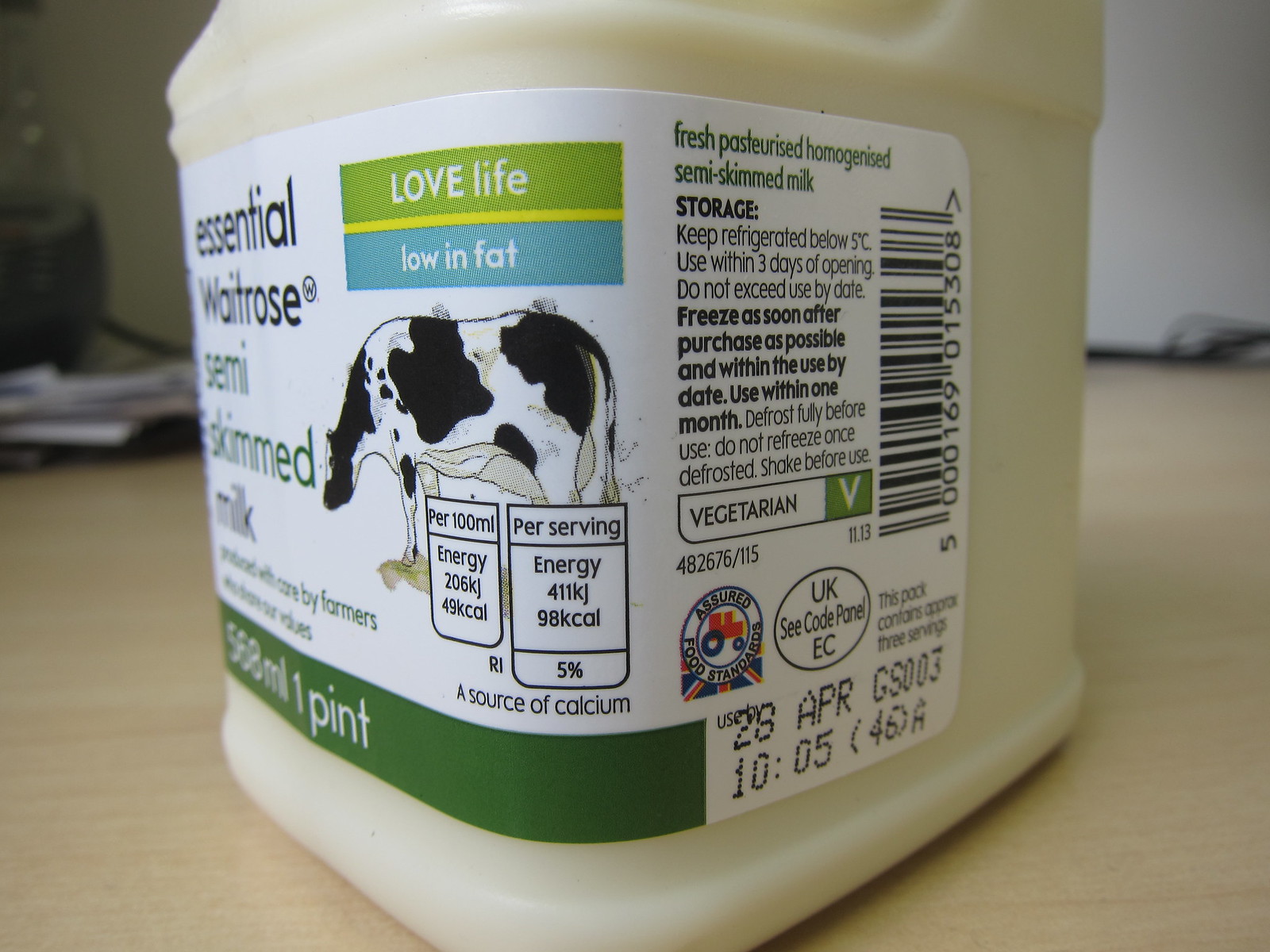This photograph showcases a pint-sized milk container, prominently labeled as "Essential Waitrose Semi-Skimmed Milk" in green text. The container itself is white, and the label features a blend of black, green, blue, red, yellow, and white text. Positioned closest to the camera, the bottle's front label comprises various detailed instructions and nutritional information. At the top-central part of the label, within a green box, are the words "Love Life," and in a blue box next to it, "Low in Fat." A black-and-white illustration of a cow is also included.

The container specifies it holds 568 milliliters, equivalent to one pint. Nutritional values are provided, indicating 206 kilojoules or 49 calories per 100 milliliters, and 411 kilojoules or 98 calories per serving, with each serving contributing 5% of the recommended daily intake for calcium. Essential additional details include an expiration date of "28th of April" and various codes like GS003. It also mentions the container holds approximately three servings.

Instructions on the label emphasize storage conditions: "Keep refrigerated below 5°C. Use within three days of opening. Do not exceed use by date. Freeze as soon as possible after purchase and within the use by date. Use within one month of freezing. Defrost fully before use. Do not refreeze once defrosted. Shake before use." Marked as "Vegetarian," this milk is certified by the United Kingdom C-Code Panel and Food Standards Assured labels.

The background of the image features a slightly out-of-focus white surface, possibly a table or floor, and some indeterminate items, adding a subtle depth to the photograph.